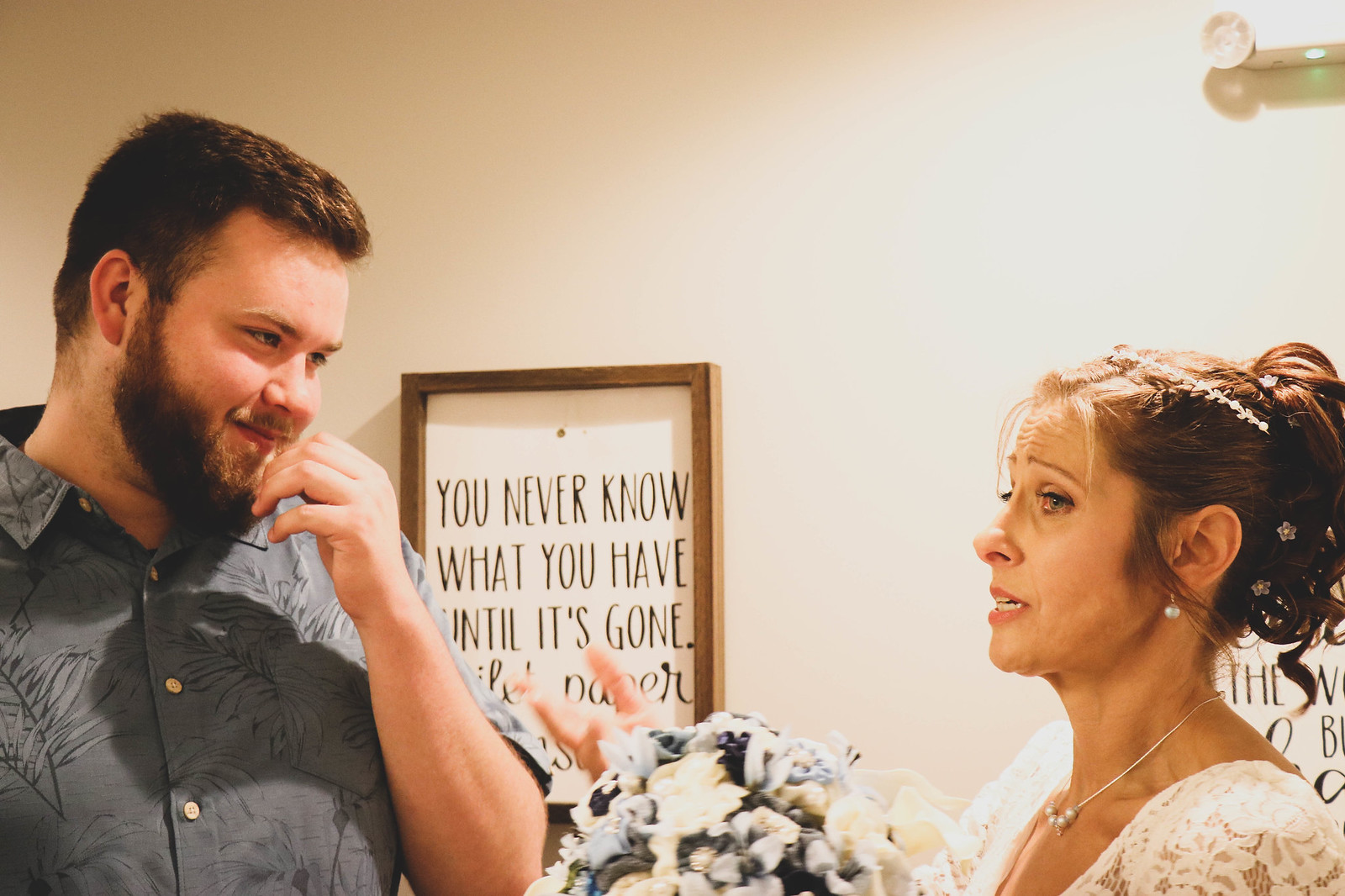The image depicts a scene that appears to be from a wedding. On the left side stands a bearded man with brown hair, clad in a short-sleeved, buttoned-up blue shirt. He is looking intently and smiling at a woman on the right, whose hair is styled up in a bun adorned with white flowers. She is dressed in a lacy white dress, accessorized with a pearl necklace and earrings. The woman is holding a bouquet of white flowers and seems to be speaking or explaining something to the man while gesturing with her right hand. They are standing in front of a whitish-tan wall that features a framed quote saying, "You never know what you have until it's gone," partially obscured by the man and the bride's hand. There is also light visible in the top-right corner of the image.